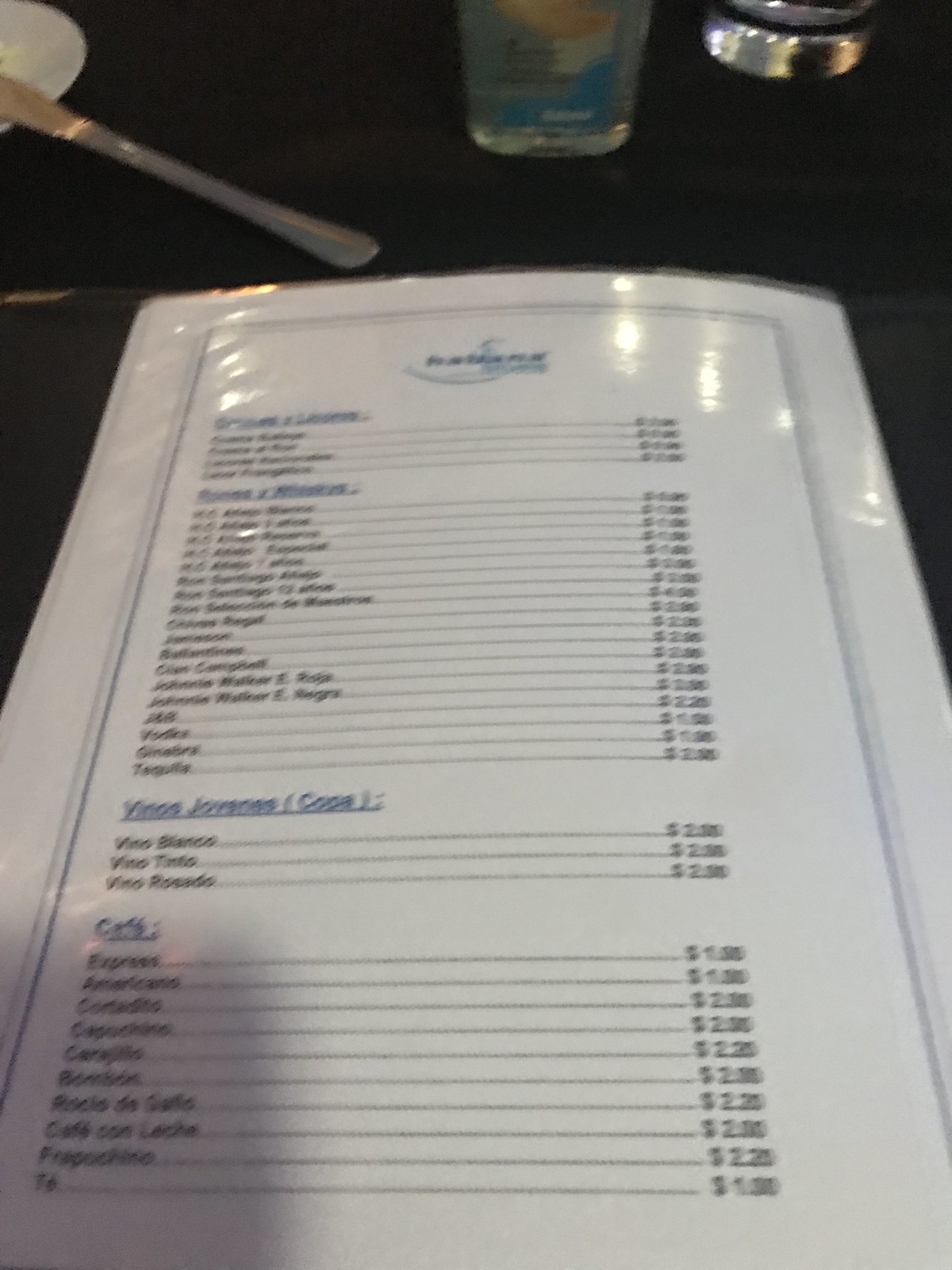This photograph captures a laminated restaurant menu sheet featuring three distinct sections, each highlighted in blue and underlined. Below each section title, the menu items are listed in black text, accompanied by their respective prices. Due to the blurriness of the image, most of the text is unreadable; however, the coffee section is somewhat discernible at the bottom. Notably, an espresso is priced at $1.00, and directly underneath, an Americano is listed for the same price. 

The menu sheet rests on a black tablecloth. In the upper left corner of the image, a white plate is partially visible. On this plate lies a silver knife. Above the plate, there is a bottle with a blue label, and to the right, only the base of a glass of water is visible.